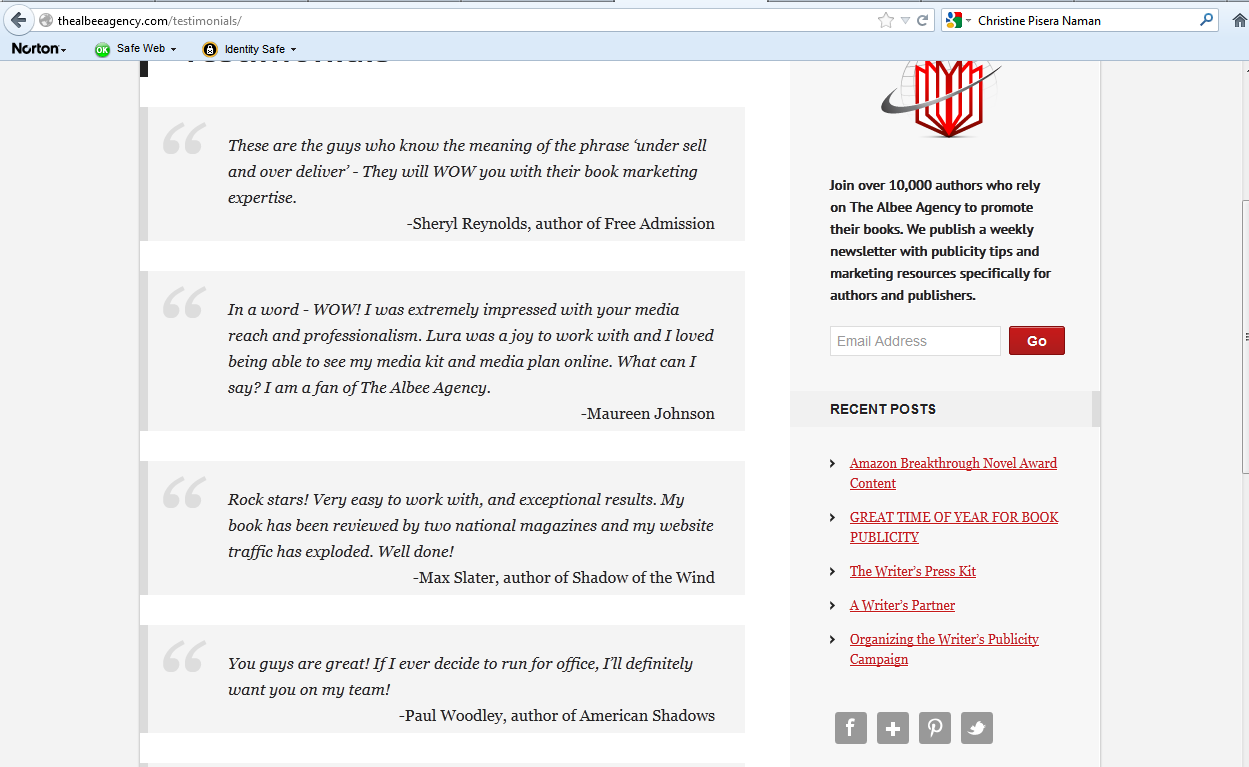This image is a screenshot from the testimonials section of the ALBI Agency's website, accessible via the URL thealbiagency.com/testimonials. The page prominently displays icons for Norton Safe Web and Norton Identity Safe at the top, indicating that these security features are active.

The main content of the page features several glowing testimonials from satisfied clients. Cheryl Reynolds, author of "Free Admission," praises the agency’s exceptional expertise in book marketing. Maureen Johnson highlights the agency's extensive media reach and professionalism. Max Slater, author of "Shadow of the Wind," commends the agency’s efforts in garnering national magazine features and increasing web traffic for his book. Additionally, Paul Woodley, author of "American Shadows," expresses his intent to continue working with the agency for future projects.

On the right side of the page, there's a promotional message encouraging authors to join the over 10,000 writers who rely on the agency’s services. This section also includes an email subscription box for their newsletter, enabling visitors to stay updated with the latest news and tips. The recent posts listed include articles such as the Amazon Breakthrough Novel Award content, advice on the optimal time of year for book publicity, tips for crafting a writer's press kit, guidance on finding a writer's partner, and strategies for organizing a writer's publicity campaign. 

At the bottom of the page, there are social media sharing icons, making it easy for users to share the agency’s offerings. The overall layout is clean and user-friendly, with a strong emphasis on client testimonials and a clear call to action for authors to engage with their services. Despite the professional appearance, there is some skepticism about the legitimacy of the website, which appears to be a WordPress site, raising questions about its authenticity and credibility.